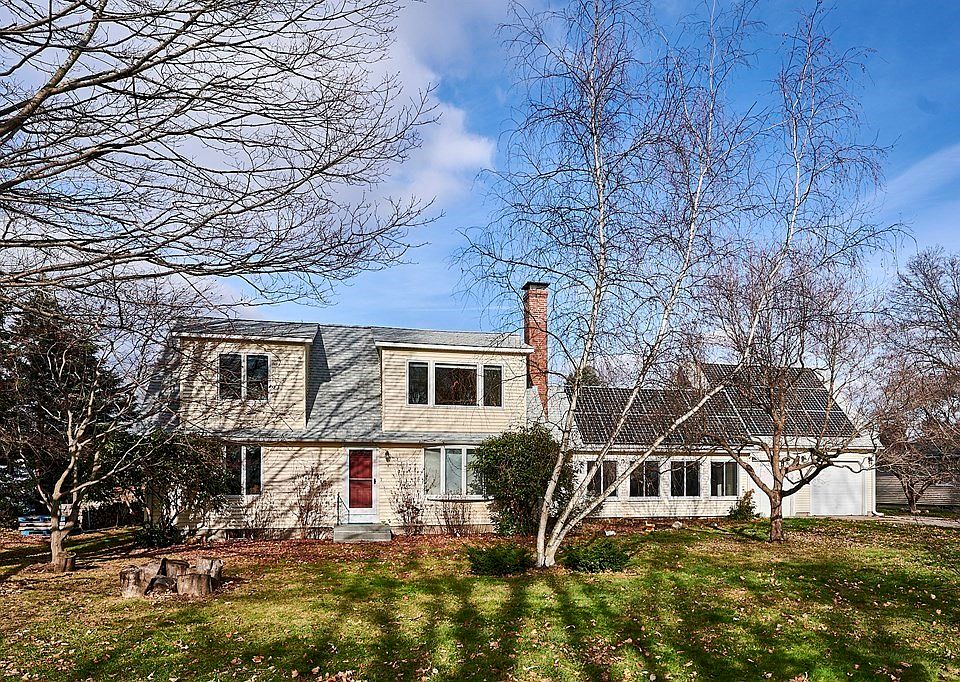This photograph captures a suburban scene featuring a prominent house with notable details and its surrounding area. The house, with its wide and two-story structure, has bone-white walls and is split into two sections. The larger section on the left features a red door with a glass storm door, flanked by bay windows that protrude from both the upper and lower floors. The right section is slightly smaller and includes a garage with two white doors. Additionally, solar panels cover the roof of this section. 

A brown brick chimney sits centrally between the two parts of the house. The house’s roof is light blue, and parts of it exhibit a distinctive curvature. In front of the house is a yard covered with patches of green grass and areas scattered with dry brown leaves, suggesting a transitional season, possibly autumn or early winter. White birch trees, some barren and others with leaves, are dispersed throughout the yard, under a blue sky adorned with white clouds. To the right side of the house, another structure is visible, contributing to the suburban ambiance of the scene.